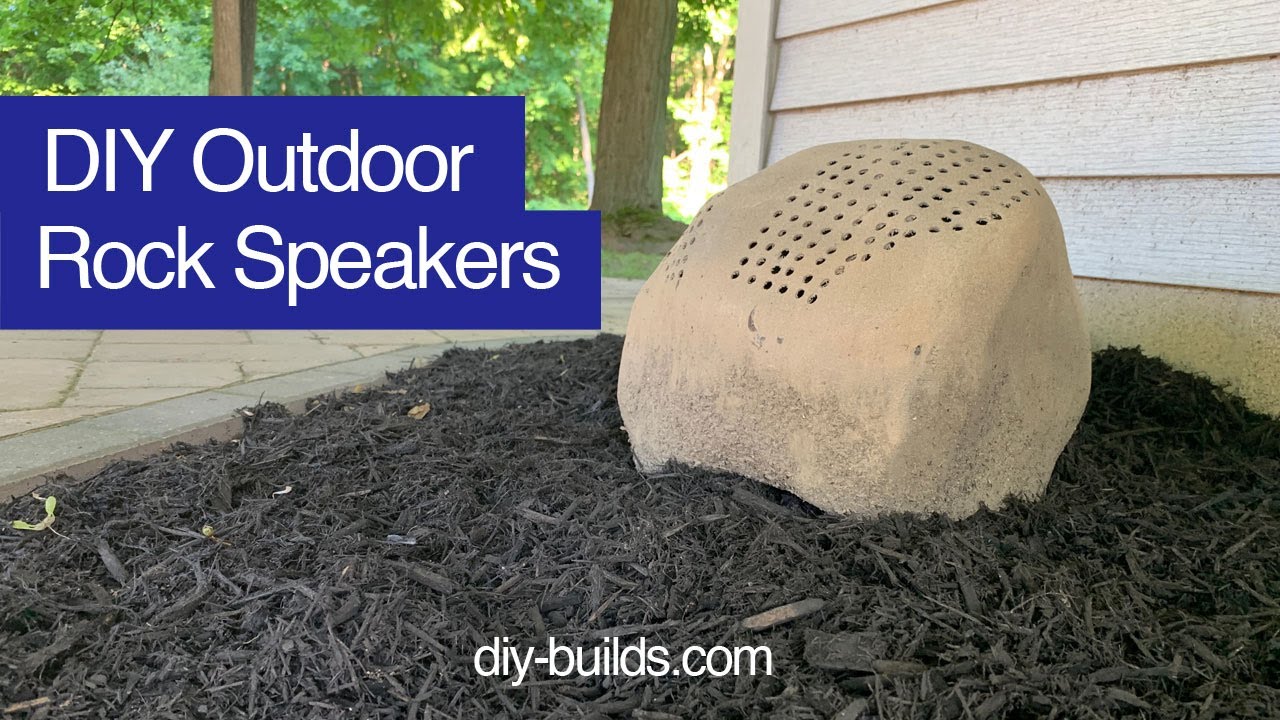This is a detailed horizontal photograph advertising DIY Outdoor Rock Speakers, prominently featuring the product name in bold white font on a purple background in the upper left corner, with the URL DIY-Build.com at the bottom center in white. The focal point of the image is a tan, sandstone-like fake rock speaker. This faux rock, designed to blend seamlessly with outdoor environments, has numerous small holes drilled into its upper portion, presumably for sound output. The speaker is positioned on dark brown, shredded wood mulch, and is surrounded by the elements of a typical backyard: a white horizontally-sided house to the right, a stone patio with pavers, and visible foliage and trees in the background. The scene is set against the backdrop of a house, emphasizing its DIY nature and intended outdoor use.